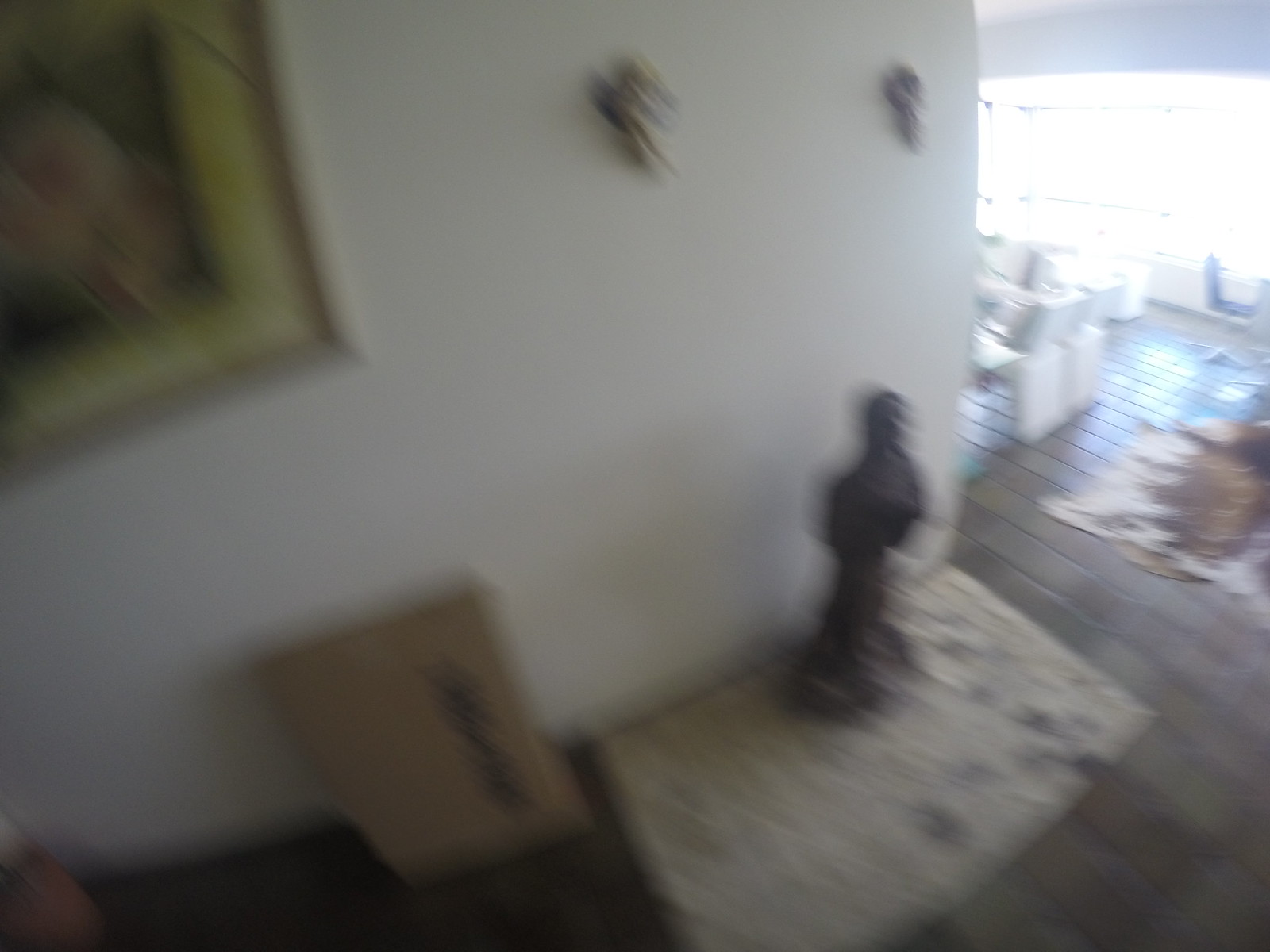This extremely blurry photograph, taken from an elevated perspective, captures the interior of a house looking down a hallway into a sunlit room. At the far right, a large, bright light filters through a massive window, casting illumination across the space. The foreground on the left reveals a white wall with several elements: a brown picture frame at the top left, two dark brown decorative pieces hanging high on the wall, and beneath them, a small, dark brown statue positioned on an off-white rug. A cardboard box leans against the wall to the left. The wooden floor stretches beneath this scene, leading to an adjoining living area. Here, a brown and white cowhide-like rug is sprawled across the floor, surrounded by two or three white couches and chairs, a blue chair, and a table, all bathed in the natural light from the window.